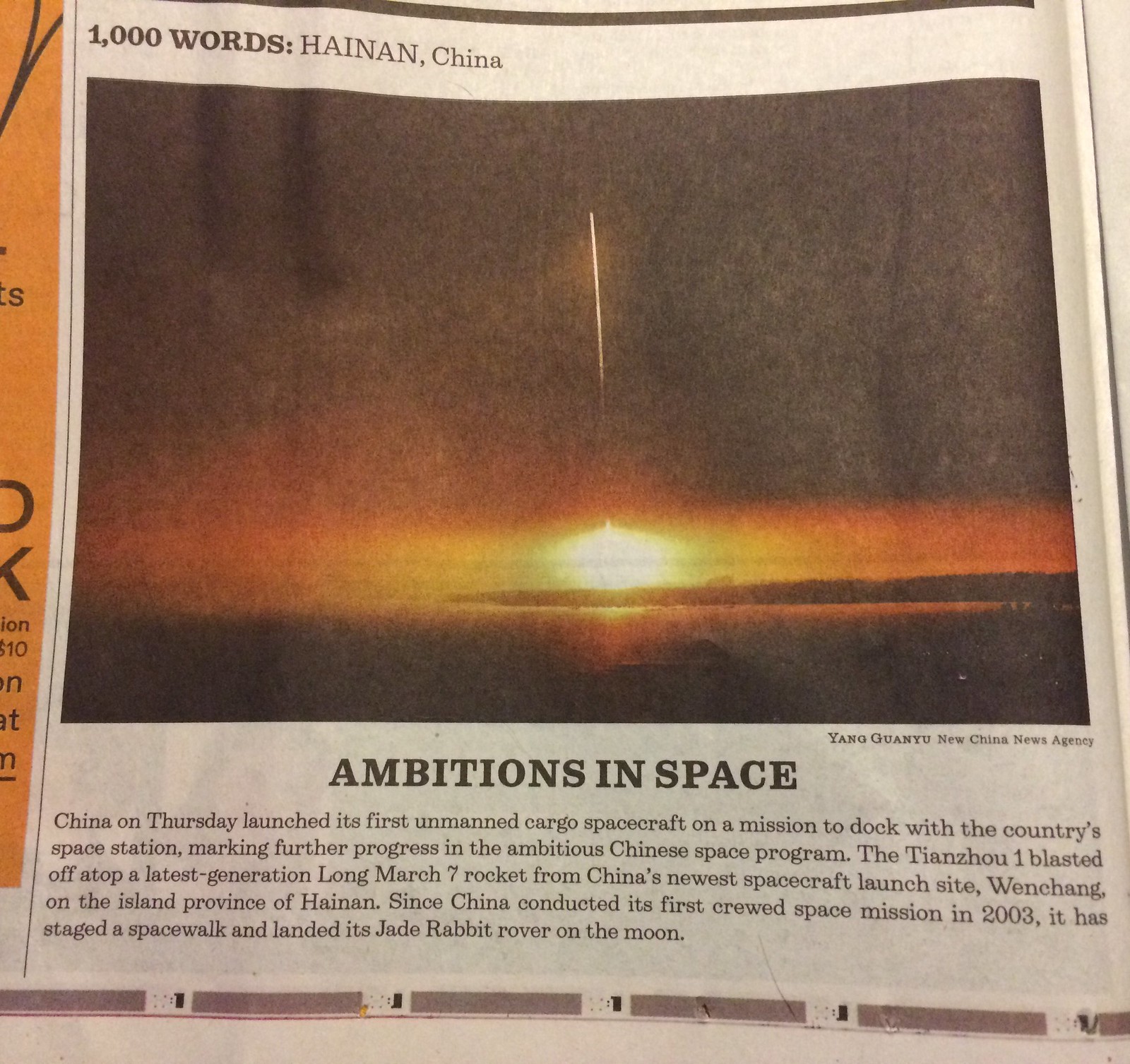The image is a detailed newspaper clipping with a single prominent object, a rocket launching into space. Dominating the entirety of the image, the text at the top reads, "1000 words, Hainan, China." The central visual depicts a rocket blasting off, surrounded by vivid colors such as tan, black, orange, yellow, white, and gray. In the lower portion of the image, the headline "Ambitions in Space" can be seen, followed by a detailed article that states, "China on Thursday launched its first unmanned